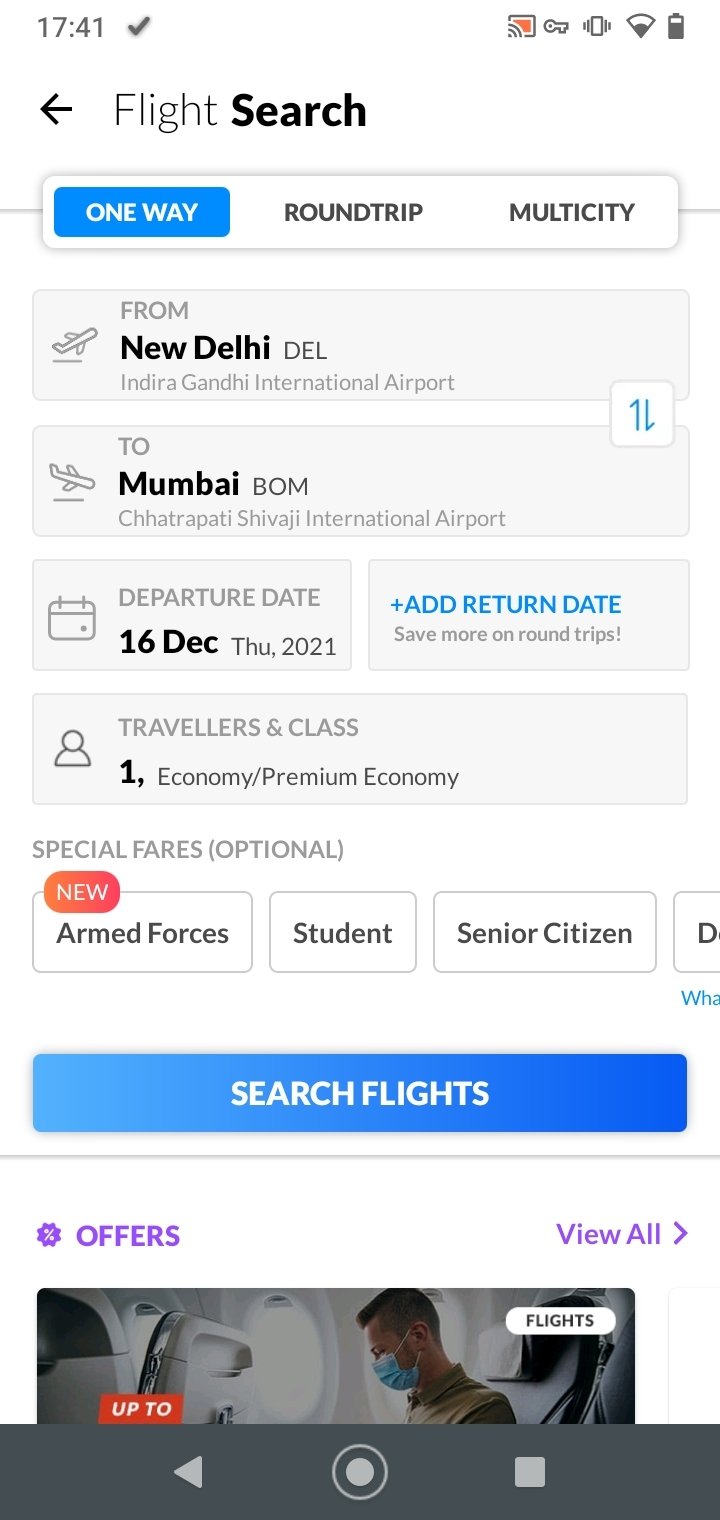This image is a screenshot captured in portrait mode, likely from a mobile phone, as indicated by the status icons. In the upper left-hand corner, the time is displayed as 17:41 alongside a checkmark, suggesting successful synchronization or an update. The upper right-hand corner features a battery icon, showing approximately 75% charge remaining.

Below this status bar, the interface primarily has a white background. At the top of this section, there is a navigation bar with "Flight Search" in bold text, flanked by a back arrow also in bold on the left side. The next row features three options for flight types: "One-way," "Round-trip," and "Multi-city." The "One-way" option is highlighted with a blue box, indicating it is currently selected.

The form begins on the next row, set against a light gray background. The departure airport is specified as Indira Gandhi International Airport in New Delhi (DEL), and the arrival airport is Chattrapati Shivaji International Airport in Mumbai (BOM).

The following section of the form is divided into two columns. On the left, the departure date is listed as December 16, 2021, which falls on a Thursday. The right column suggests adding a return date to save more on round trips.

Further down, there are options for traveler count and class selection: "1 traveler, Economy." Additional special fare options are listed, including "Armed Forces," "Student," "Senior Citizen."

A large, light blue button is displayed prominently, labeled "Search Flights."

Below the search button, there's a section with offers. On the left, the word "Offers" is displayed in purple, and on the right, a "View All" button is available. The lower part of the screenshot shows the top half of an airplane image, depicting people inside the airplane.